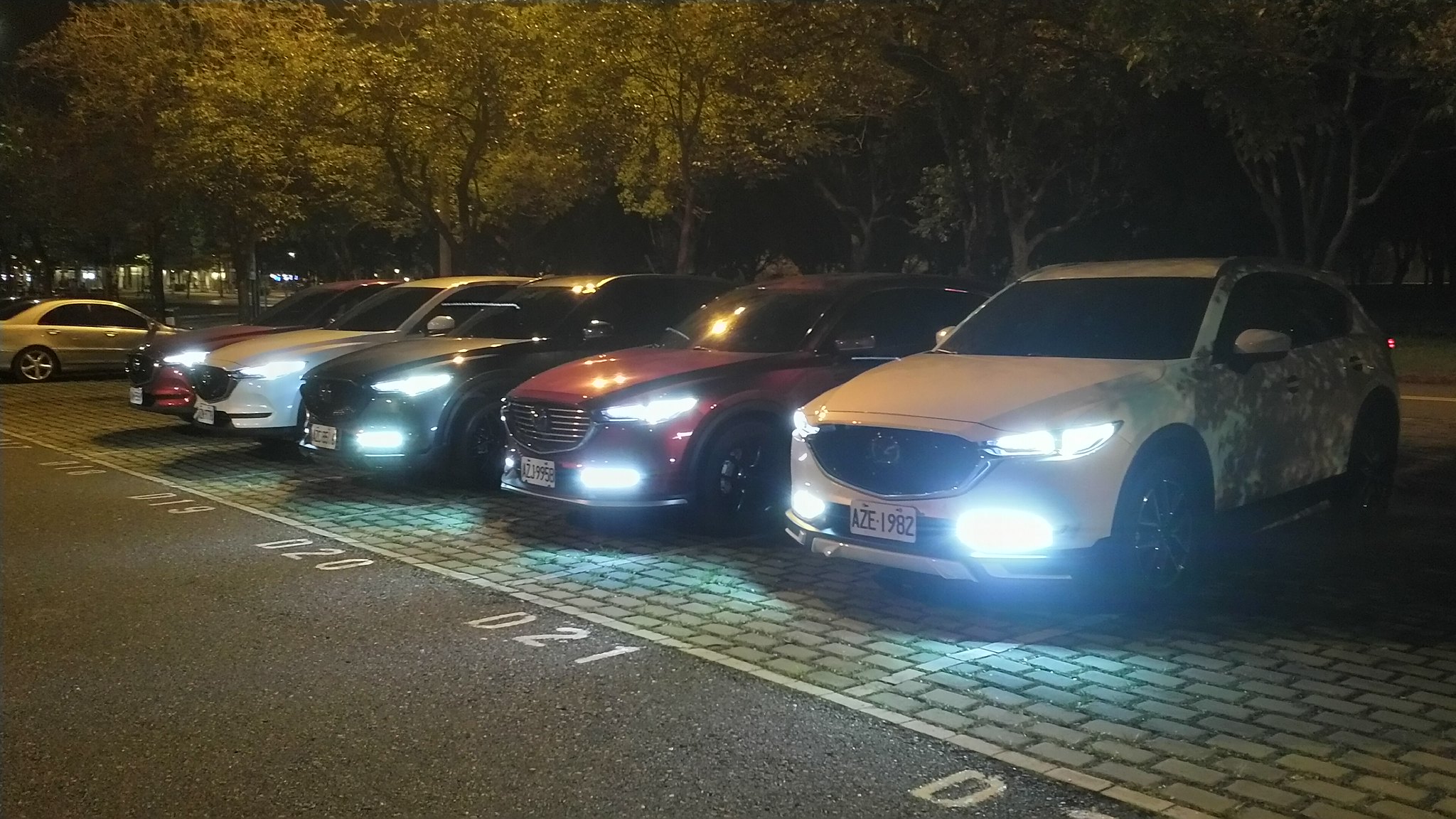This nighttime exterior photograph captures a line of five vehicles, all with their headlights illuminated, backed into parking spaces delineated by white lines on a brick surface interspersed with either short grass or dirt. The foreground transitions into asphalt, on which parking space numbers like D18 to D22 are marked. Closest to the camera, the vehicles appear to consist of a white SUV, a maroon SUV, a dark gray or possibly black SUV, another white SUV, and a red hatchback, although the exact colors may vary slightly. To the side and further back, there is another vehicle, possibly yellow, parked in the opposite direction. Light from a nearby parking lot lamp in the upper left corner casts an ambient glow over a dense line of trees that frame the background. The scene is dominated by the white headlights and potentially fog lights, which illuminate the immediate surroundings.